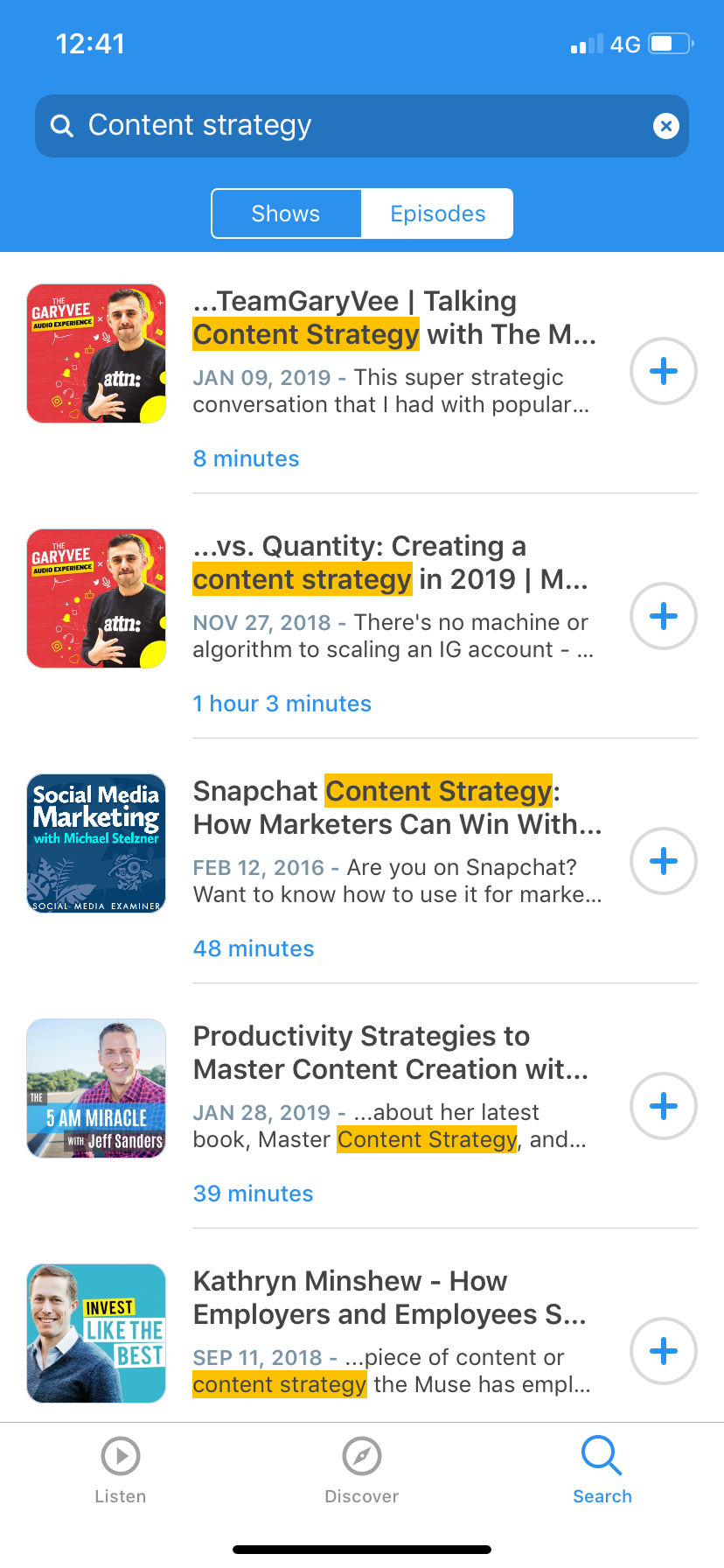This is a detailed screenshot taken from a mobile phone. In the upper left-hand corner, the time is displayed as 12:41. On the upper right-hand corner, a signal strength icon indicates two out of five bars, followed by the label "4G", and a battery icon showing approximately half charge. The browser or app window displays search results for "content strategy". Several results are visible, including:

1. "Team Gary V talking content strategy with the M" - A strategic conversation featuring a popular figure.
2. "This one's eight minutes versus quantity: Creating a content strategy in 2019" - Dated November 27, 2018.
3. "There's no machine or algorithm to scaling an IG account" - A video lasting one hour and three minutes.
4. "Snapchat content strategy: How marketers can win with" - An inquiry on leveraging Snapchat for marketing, lasting 48 minutes.
5. "Productivity strategies to master content creation" - Discussing the latest book "Master Content Strategy" by Catherine Minshew, focusing on the intersection of employers, employees, and content strategy.

The last line of the screenshot is cut off, ending with "the news has".